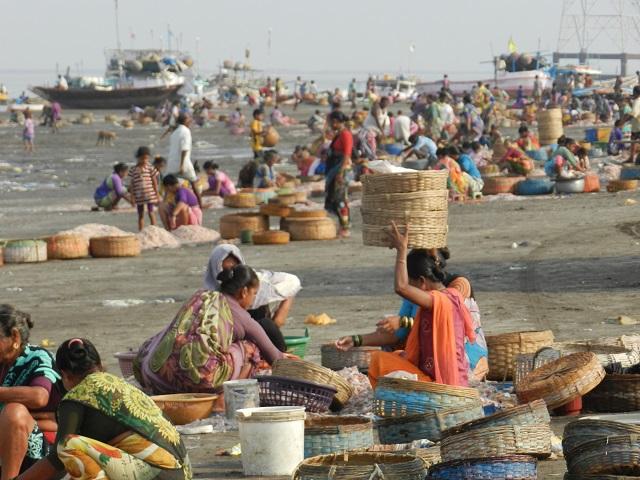This vibrant, color photograph captures a bustling seaside market scene set on a sandy shoreline. The foreground features a group of women, predominantly adorned in colorful attire, surrounded by numerous round baskets. Among them, a woman stands out on the right, wearing an orange sari over a pink, short-sleeved t-shirt, impressively balancing four baskets on her head. Around her, three other women are engaged in picking and placing grains into their own baskets. Scattered on the ground in the foreground and stretching into the background are more baskets, suggesting a thriving market environment. Children can be seen playing, adding a lively dynamic to the scene. The backdrop is equally crowded with people and is punctuated by ships and the ocean, with the gray sky adding a serene contrast to the busy activity below. The photograph offers a detailed snapshot of daily life in this seaside community, capturing both the commerce and the communal spirit of the place.